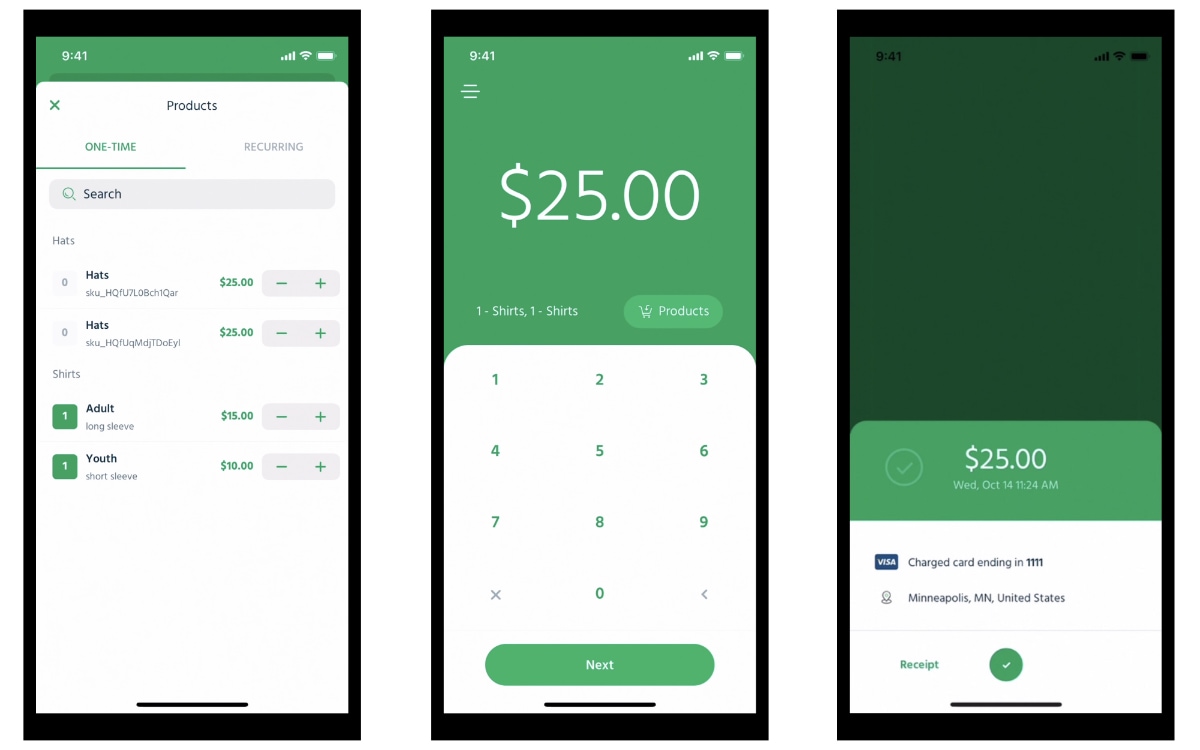Three sequential phone screenshots detail the process of making a purchase:

1. The first screenshot displays a mobile shopping page with a green status bar denoting the time as 9:41 AM, full battery, and good internet connectivity. At the top, it shows a section labeled "Products" with options to make it a one-time purchase or a recurring order, currently set to "one-time." Below is a search bar, and underneath that, two types of hats are listed, each priced at $25. The display allows users to add or subtract items using plus or minus buttons for each product. Following the hats, there are shirt categories—adult shirts priced at $15, and youth shirts with respective plus or minus buttons for quantity adjustment.

2. The second screenshot presents what appears to be a calculator interface or the checkout page where quantities and items are finalized. It indicates an order of "one shirt" and "one shorts," with sections for "Products" and numerical input. A "Next" button is also visible for proceeding with the order.

3. The final screenshot confirms the purchase details: a successful transaction of $25, dated Wednesday, October 14th at 11:24 AM. It also notes the payment method, a Visa card with the card number partially obscured, and the transaction location listed as Minneapolis, Minnesota, United States. The screen includes a receipt confirmation and a checkmark indicating approval of the purchase.

The detailed progression from product selection to payment confirmation encapsulates a smooth shopping experience on a mobile device.